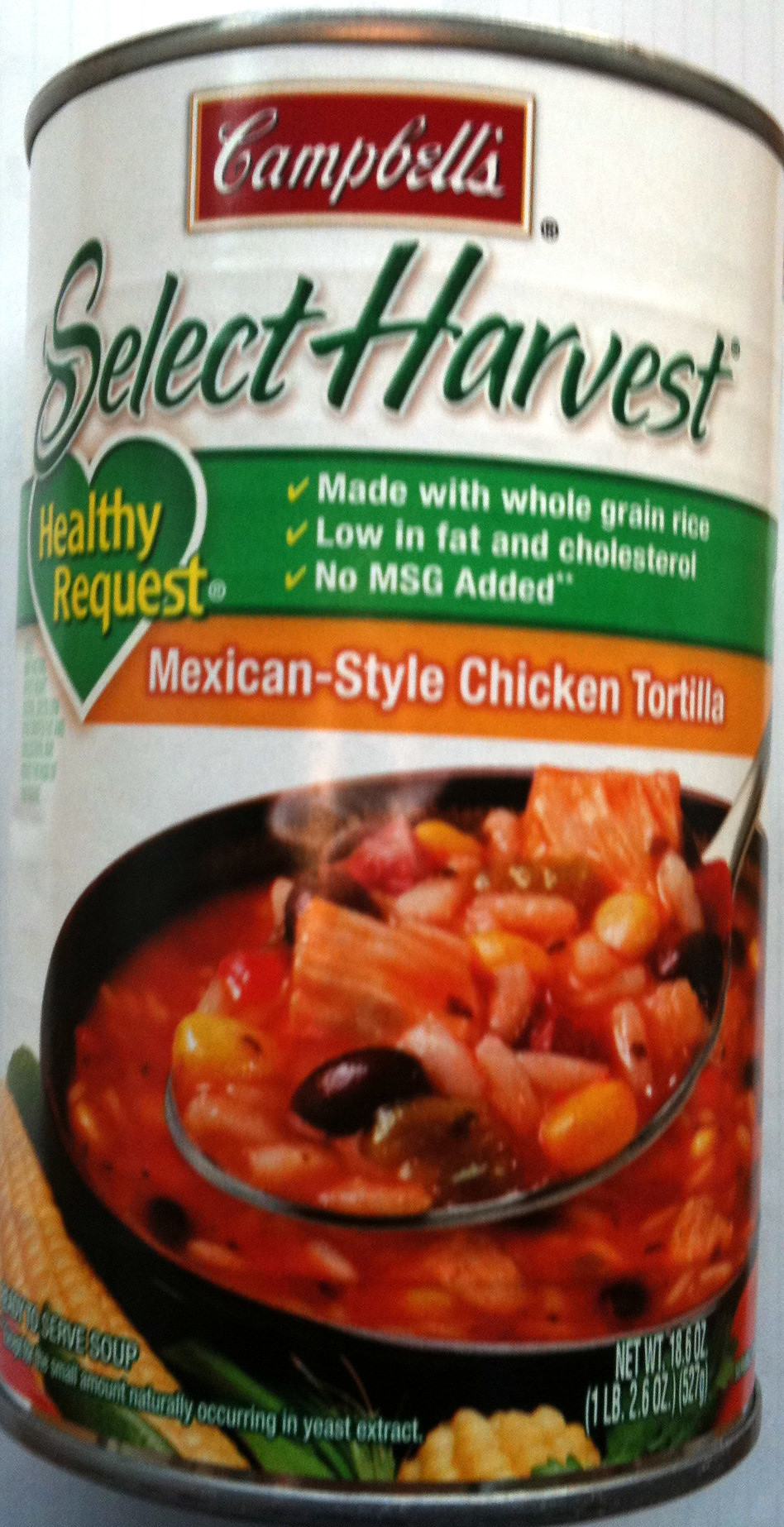This is a detailed image of a Campbell's soup can, prominently featuring various elements on its label. At the top, a red square displays the iconic "Campbell's" logo in white letters. Just below, "Select Harvest" is written in green font, leading down to a green heart with "Healthy Request" inscribed in yellow letters. To the right of the heart, three yellow check marks accompany the phrases: "Made with Whole Grain Rice," "Low in Fat and Cholesterol," and "No MSG Added."

Continuing downward, an orange banner announces the soup flavor: "Mexican Style Chicken Tortilla." Additional information at the bottom states the weight as "Net WT 18.6 ounces (1 pound, 2.6 ounces)."

The central image is a black bowl filled with a vibrant red chili, steaming hot, and shown with a spoonful being lifted. The chili contains black beans, rice, corn, and various seasonings, with yellow corn on the cob also depicted near the bowl. The label background transitions from white at the bottom to more colorful elements around the text and imagery, creating a visually appealing layout. The aluminum can itself has a metal top and bottom, completing the classic Campbell's look.